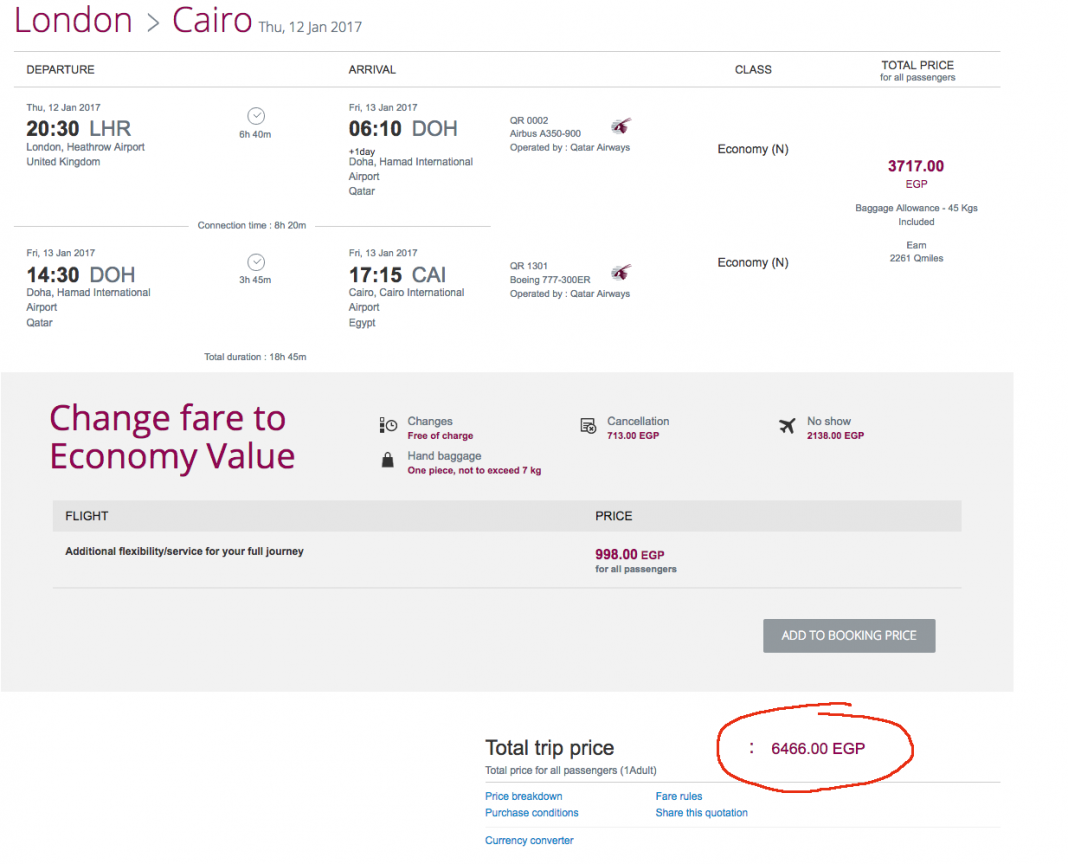Detailed Caption:
---

This image depicts an itinerary page detailing a flight from London to Cairo. In the top left corner, the heading "London to Cairo" is prominently displayed in magenta text. Directly beneath this title, the date "Thursday, 12 Jan, 2017" is written in smaller text. 

Below the header section, the itinerary layout is divided into columns labeled "Departure," "Arrival," "Class," and "Total Price."

Under the "Departure" column, the first flight is listed for "Thursday, 12 Jan, 2017," with a departure time of "20:30" from "LHR - London Heathrow Airport, United Kingdom." 

To the right of the departure time, an arrow indicates the flight duration of "6 hours and 40 minutes."

Following this, the "Arrival" column notes that the flight will arrive on "Friday, 13 Jan, 2017," at "06:10" in "DOH - Doha Hamad International Airport, Qatar," also marked with a "+1 day" to account for the overnight travel.